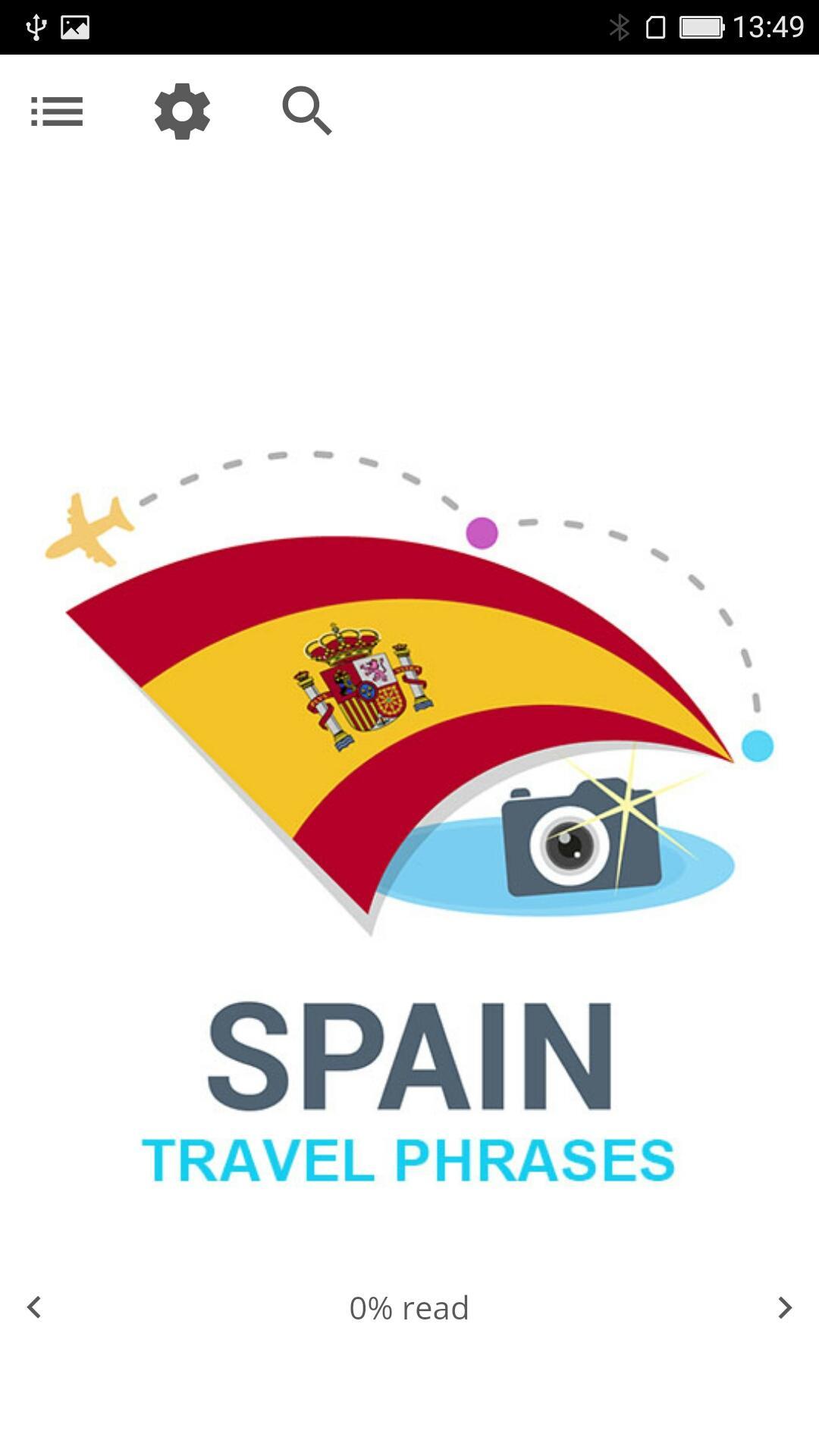The image is a screenshot taken from a non-iPhone smartphone, discernible by the distinct user interface. At the very top left corner, there is a series of small icons. The first appears to be a symbol resembling a trident or Bluetooth, followed by what seems to be an image icon. To the right of these, there's a Bluetooth icon which is turned off, a piece of paper icon, and a full battery icon indicating 100% charge. The time displayed is 13:49 in military time, corresponding to 1:49 PM.

Directly below these icons, on the far left, there is a menu button that is not currently opened. Proceeding to the right, next to the menu button is a gear icon representing the settings, and further right is a search bar.

Beneath these interface elements, the main content of the screenshot features an image that catches the eye. It depicts the flag of Spain, albeit slightly distorted. Overlapping this flag is a camera submerged in a pool of water, seemingly capturing an image of the flag. Above the flag, there are graphics of an airplane, colored yellow, following a route marked by dotted lines, moving between two points—one blue and one purple—signifying two destinations.

Below the image, the text "Spain travel phrases" is prominently displayed in blue. This section appears to be part of a digital book or pamphlet, indicated by the text "0% read." Additionally, navigation arrows are present on the left and right sides, suggesting that the user can flip through the pages.